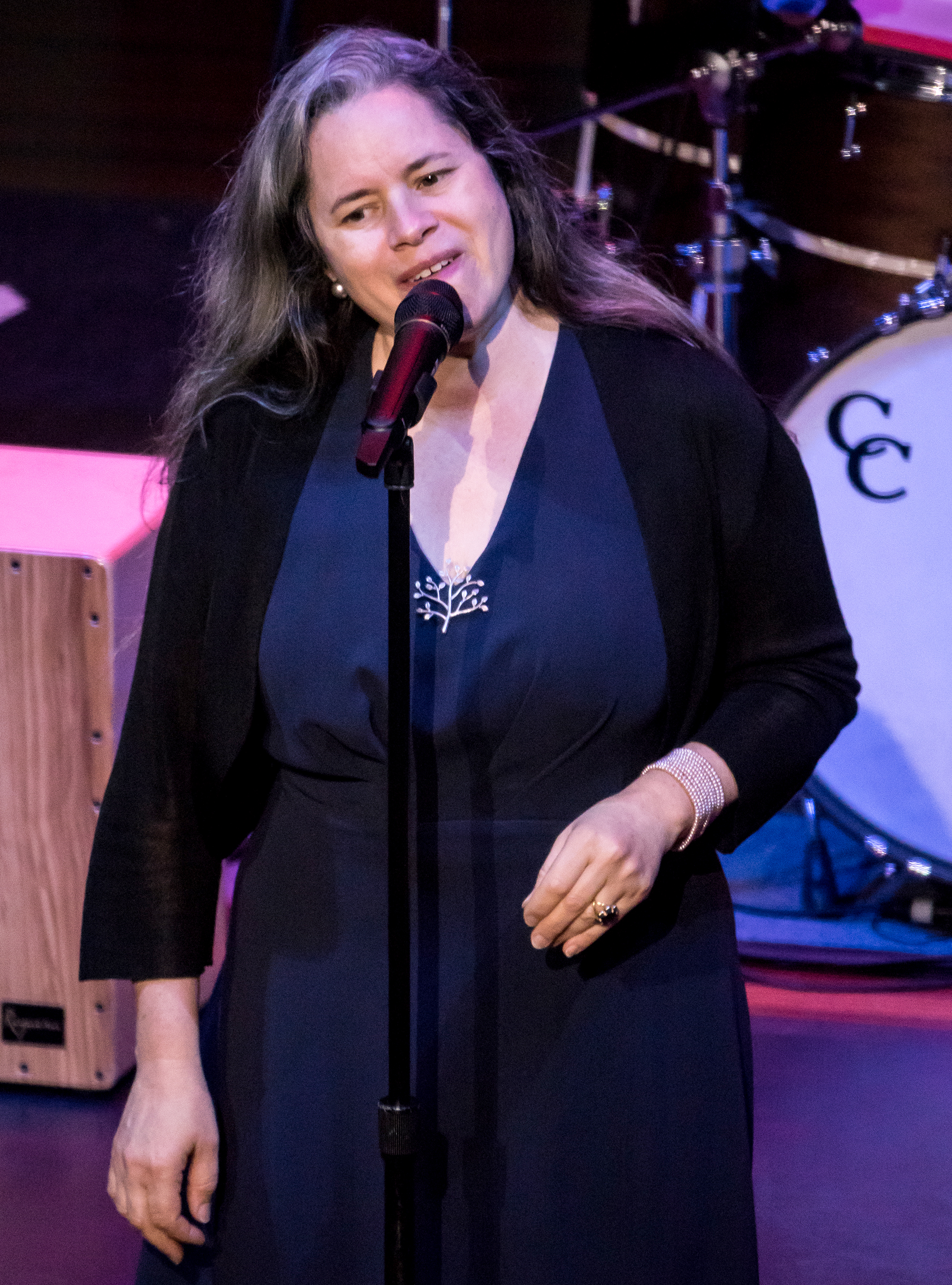In this close-up photograph, a woman is captured singing into a black wireless microphone, her head slightly tilted to the left. She is dressed in a dark blue v-neck dress adorned with a black sweater jacket over it. A delicate white pendant, shaped like a tree with intricate branches, rests on her chest. Her left arm hangs loosely by her side, displaying a ring on her ring finger and a light tan bracelet with small beads around her wrist. In the background, a drum set is partially visible, including a large white drum inscribed with "CC," set against a purple stage floor. To her left, a wooden block, likely part of the stage equipment, is also visible.